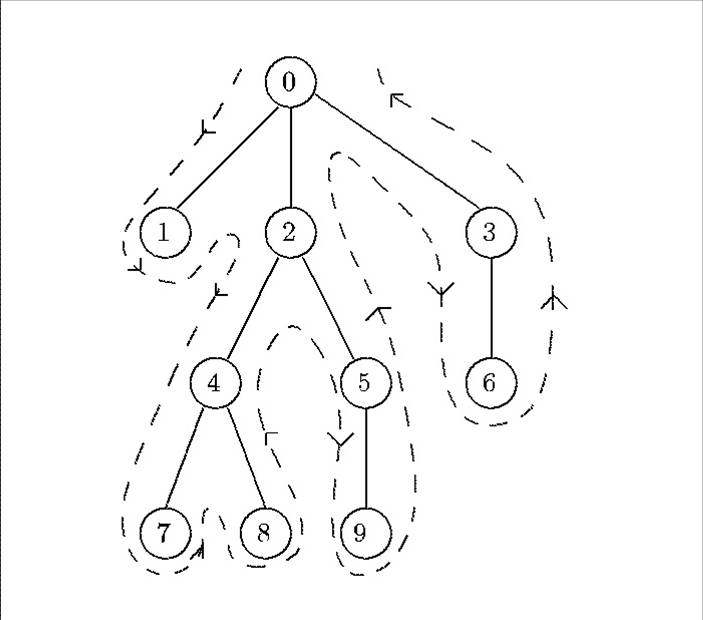A detailed diagram of a non-conventional maze is depicted against a white background. The maze comprises both solid and dotted lines, all rendered in a dark grey color. The solid lines are sequentially numbered from 0 to 9, while the dotted lines feature arrows indicating the direction you are supposed to follow. However, the path marked by these arrows does not proceed in a straightforward numerical sequence; instead, it traverses through the numbers in a seemingly random order: 0, 1, 2, 4, 7, 8, 5, 9, 6, 3, and finally to the finish. The overall design of the maze does not resemble any specific shape, although it may initially give the impression of a human figure upon first glance. Closer inspection reveals a more intricate and abstract pattern, defying easy categorization.